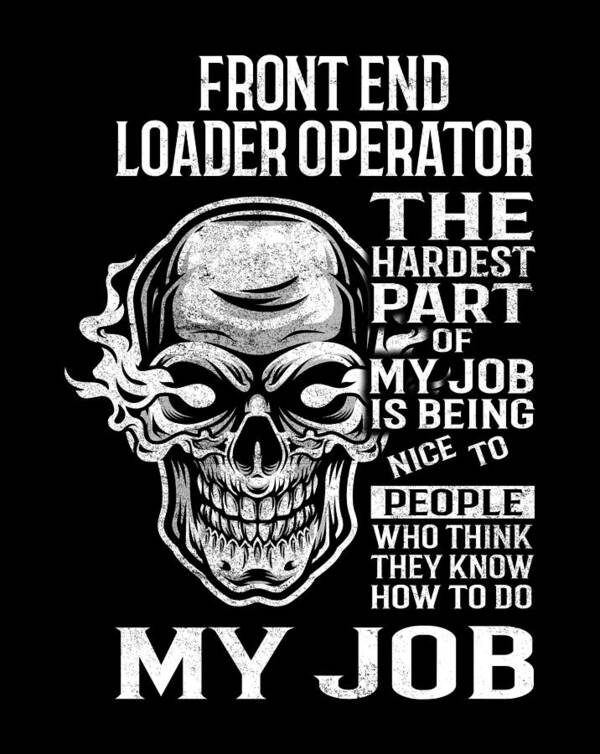This poster, set on a black background, features a bold and somewhat gritty white/gray text that reads at the top: "Front End Loader Operator" in large letters. Below this heading, aligned to the right side, is a list of phrases describing a sentiment many might relate to: "The hardest part of my job is being nice to people who think they know how to do my job." The prominent phrase "my job" is emphasized in large, striking letters across the bottom of the poster. Dominating the left side and partially overlapping with the text is a vivid, detailed graphic of a skull. This skull, depicted in shades of gray with white accents, boasts fiery flames bursting from its eye sockets and extending around the back of the head. The skull also features a nose ring and tightly clenched teeth in both the upper and lower jaws. This intense image amplifies the overall fierce and edgy tone of the poster.